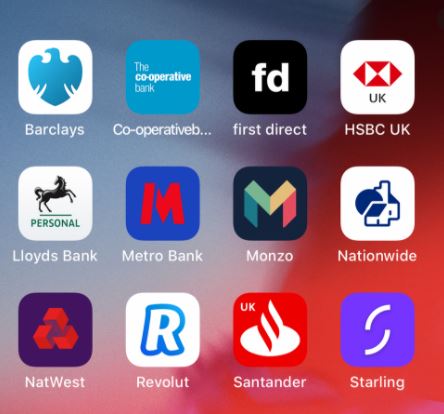The image presented is a square-shaped screenshot of a smartphone's home screen displaying a grid of financial app icons, structured in a 4x3 arrangement. Starting from the upper left corner, the first icon is for Barclays, featuring a blue bird transitioning from a medium blue to a darker blue. Next is the Co-operative Bank app, identified by the partial text "Cooperative" and "E..." along with a medium blue background and a white shopping bag logo.

On the second row, the first app is First Direct, represented by a black background with "FD" in white letters. Following it is the HSBC UK app, showing a white background with a horizontal red diamond and the letters "UK" beneath it. The third icon is for Lloyds Bank, displaying an image of a horse above the word "Personal." Concluding this row is the Metro Bank app, marked by a red "M" on a blue background.

Descending to the third row, the first app is Monzo, characterized by a black background and a multicolored "M." Next is the Nationwide app, featuring a small blue house icon. The final app is NatWest, symbolized by a logo that resembles a red recycling sign.

Each icon is clearly distinguishable, featuring unique color schemes and logos representative of their respective banking institutions.